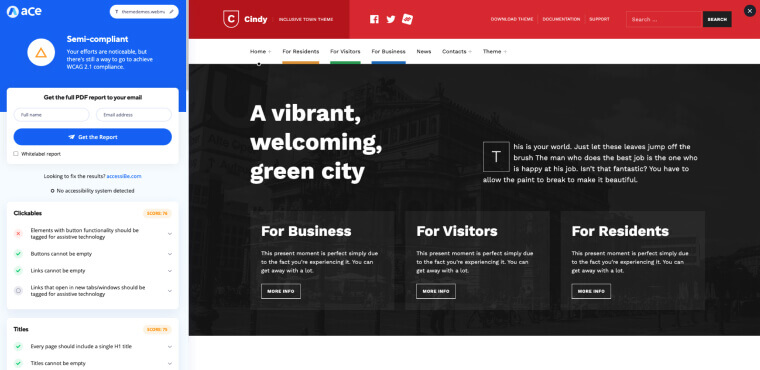A detailed screenshot of a web page is shown. On the left-hand side, there is a vertical sidebar. At the very top of this sidebar is a blue field that prominently displays the acronym "ACE" in white letters. Below "ACE," the words "semi-compliant" are written. Further down, there is a section of text that is too small to be legible. Directly beneath the blue field, a white field is visible, which appears to contain a search bar along with some menus.

Occupying the larger part of the image is the main page content, positioned to the right of the sidebar. At the top of this section, there is a horizontal red stripe featuring the name "Cindy" in white text. This red stripe also includes additional white menu text that is too small to read clearly. Below this red stripe, another horizontal stripe appears, this time in white, which seems to serve as the primary navigation menu. The menu options read "Home," "For Residents," "For Visitors," and "For Business."

Further down the main page is a prominent black area with the slogan "A Vibrant Welcoming Green City" written in white text. Below this slogan, there are several lighter black squares arranged in a grid-like fashion. These squares are labeled as follows: "For Business," "For Visitors," and "For Residents."